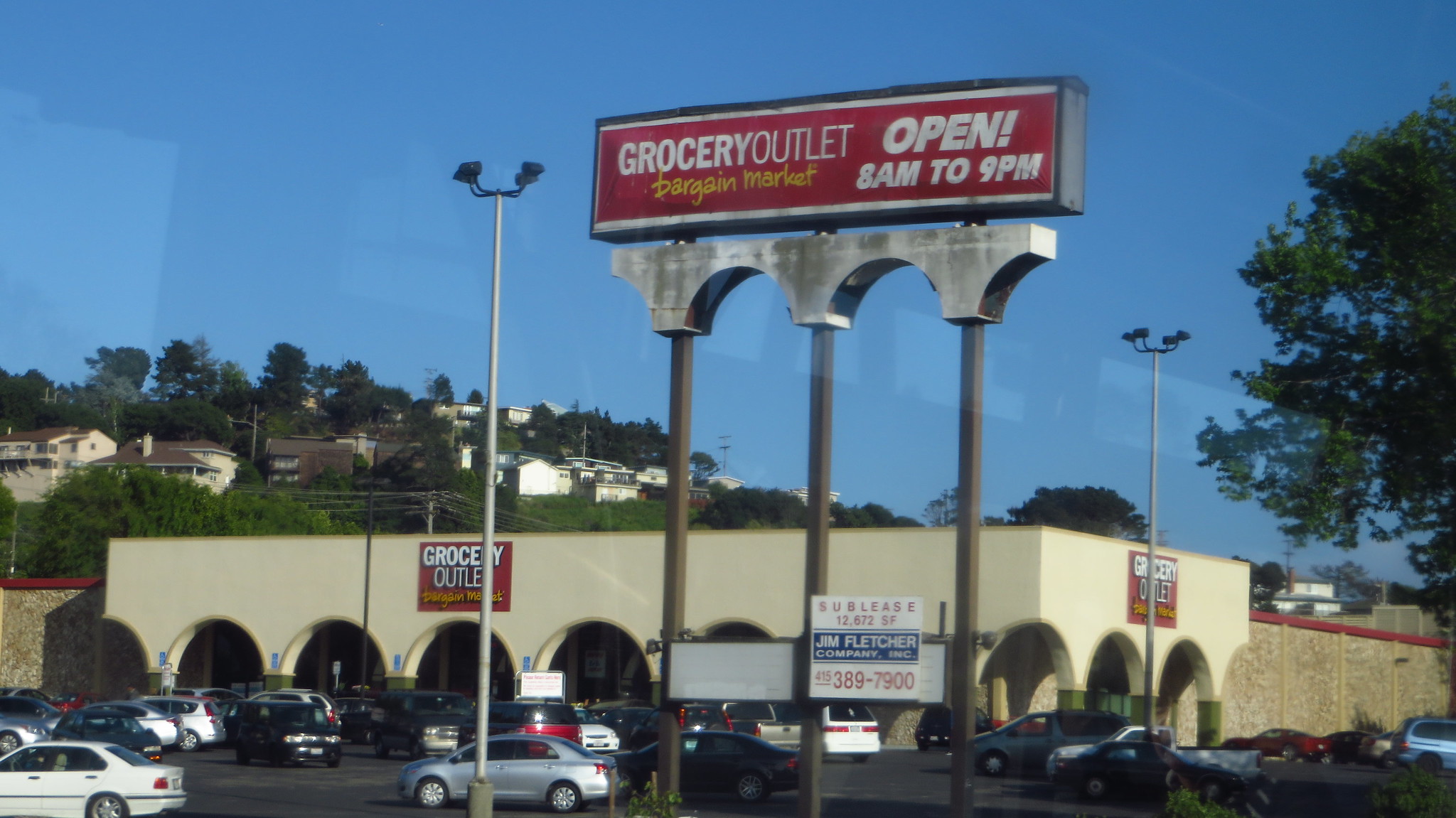In this rectangular, horizontally longer photograph, we see an outdoor scene on a clear, blue-skied day, depicting a slightly lower-income area. The focus is on a large grocery store named "Grocery Outlet," identifiable by a prominent sign that reads, "Grocery Outlet Open 8 a.m. to 9 p.m., Bargain Market." This sign is supported by three large metal columns above the store's entrance. The parking lot in front of the store is filled with numerous cars, indicative of a busy day. There are two tall streetlights providing illumination to the parking area. To the right of the image and in the upper left corner, green trees enhance the scene's natural beauty. In the upper left corner, the horizon meets a tree-lined area dotted with homes on a hill, adding depth and a sense of community to the photograph.